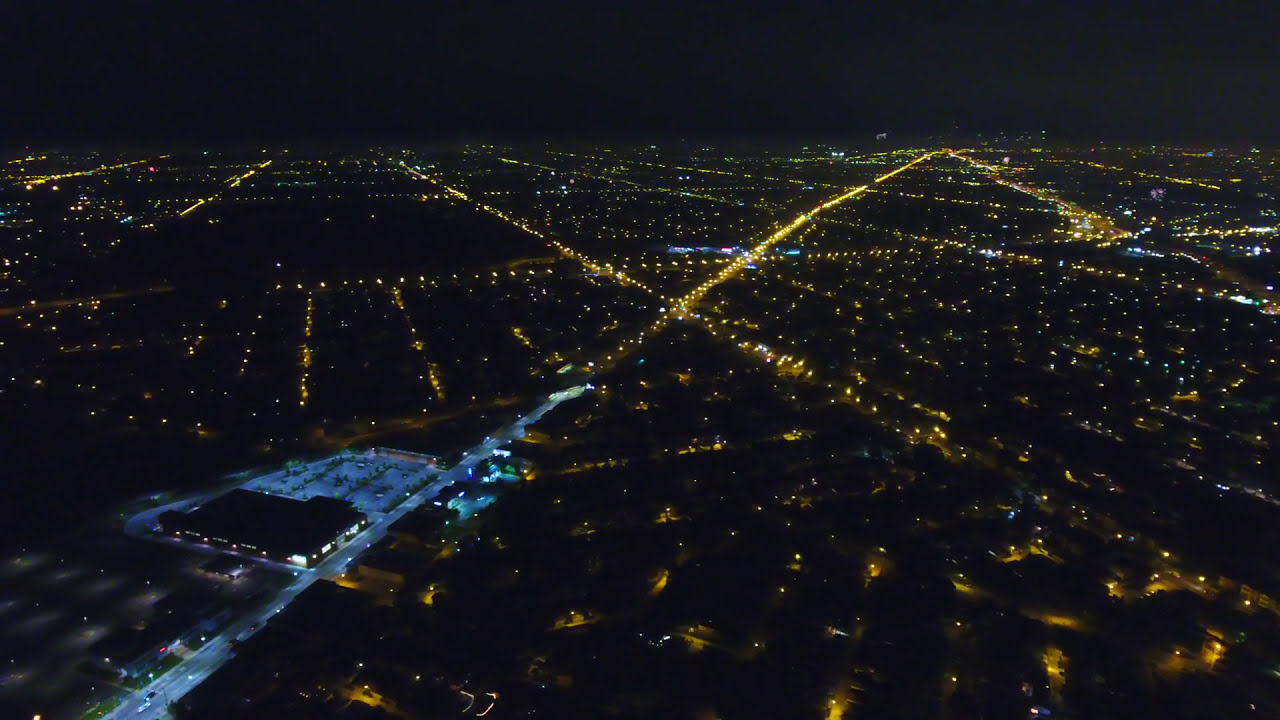This aerial, nighttime photo captures a city's intricate grid of illuminated roads and square blocks. Taken from a high altitude, likely from an airplane, the cityscape is outlined by an array of lights that pierce through the encompassing darkness. The scene below is dominated by the crisscrossing network of streets, dotted with the glow of car headlights and street lamps that cast a warm yellow-orange hue. A notable feature in the lower left corner is a retail center with two buildings and a central parking lot, distinguished by a striking blue tint from energy-efficient lights, contrasting with the surrounding yellowish street lights. Far in the distance, a concentration of brighter lights suggests a bustling downtown area, providing a vibrant focal point in the vast expanse of night.